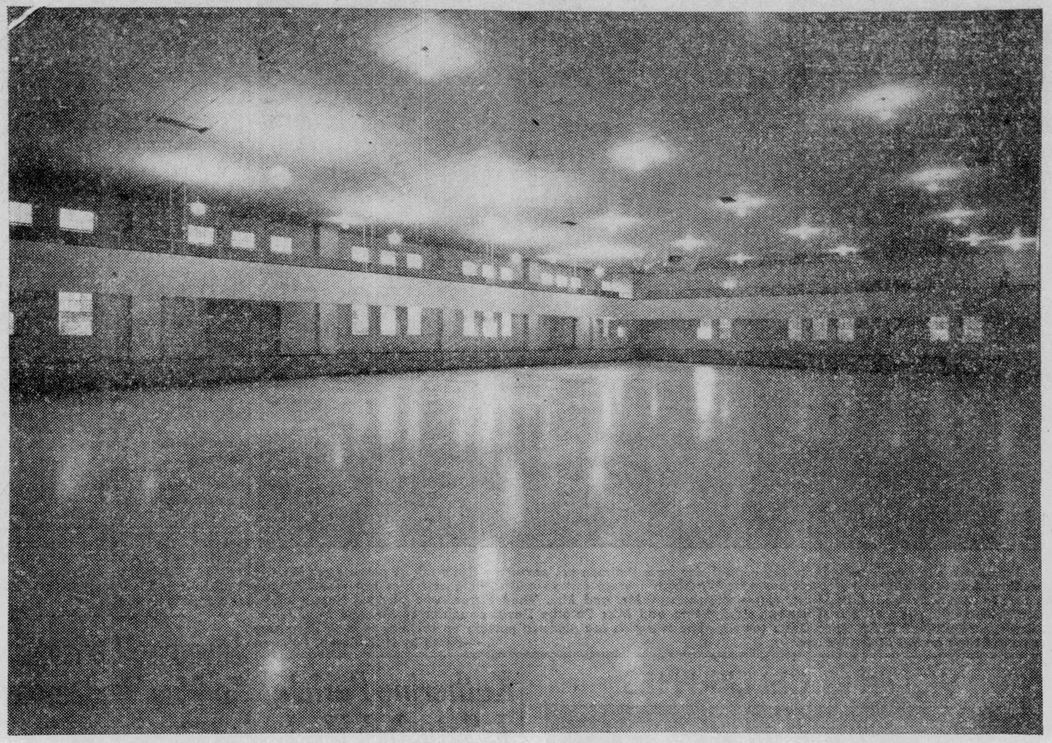In this extremely grainy, black-and-white photograph of a large, open indoor room, the artificial light and square format are apparent. The slick, possibly wooden or cement floor reflects the ceiling lights that are arrayed in rows throughout the dark-colored ceiling. The right-hand side of the room features a wall that extends across and corners just right of the center, potentially indicating another section of the room. Along the walls, there are two rows of windows: one at a normal height above the floor and another set higher up. Between these windows runs a horizontal ledge or wood piece. Despite the room’s vastness and openness, akin to a gymnasium or an ice arena, no sporting equipment such as basketball nets or courts is visible. The photograph is characterized by its hazy, dark quality, making additional details difficult to discern. The image itself is framed by a thin, grey border, enhancing its stark, minimalist aesthetic.